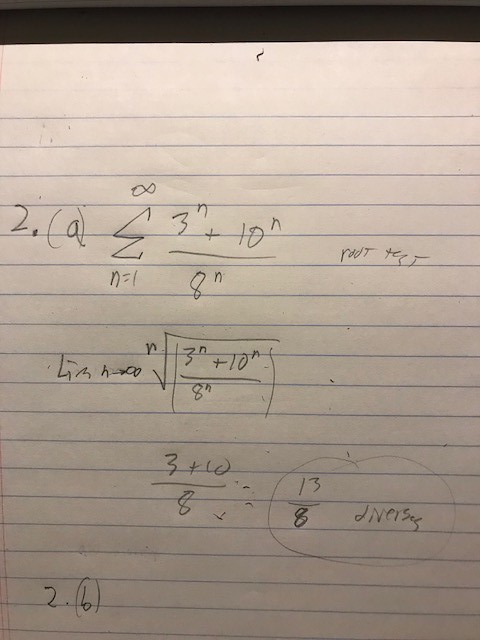A photograph features a piece of lined notebook paper, showcasing a slightly off-white color with distinct blue horizontal lines. Positioned at the top of the image, a black strip suggests the surface on which the paper rests. The notebook page displays handwritten calculus formulas in the upper section, including a notation resembling "A/Q," followed by a summation symbol (Σ) with limits from n=1 to infinity. The accompanying formula is written as (3^n + 10^n) / (8^n). To the right, the term "Root Test" is visible.

Further down, on the lower portion of the page, the notation "LIM" is evident, likely indicating a limit in mathematical terms. Below this, an expression shows "H → ∞" next to a square root symbol. Under the radical, enclosed by vertical lines, is the formula (3^n + 10^n) / (8^n). Additional complex mathematical expressions appear scattered throughout the page, conveying an intense focus on calculus concepts.